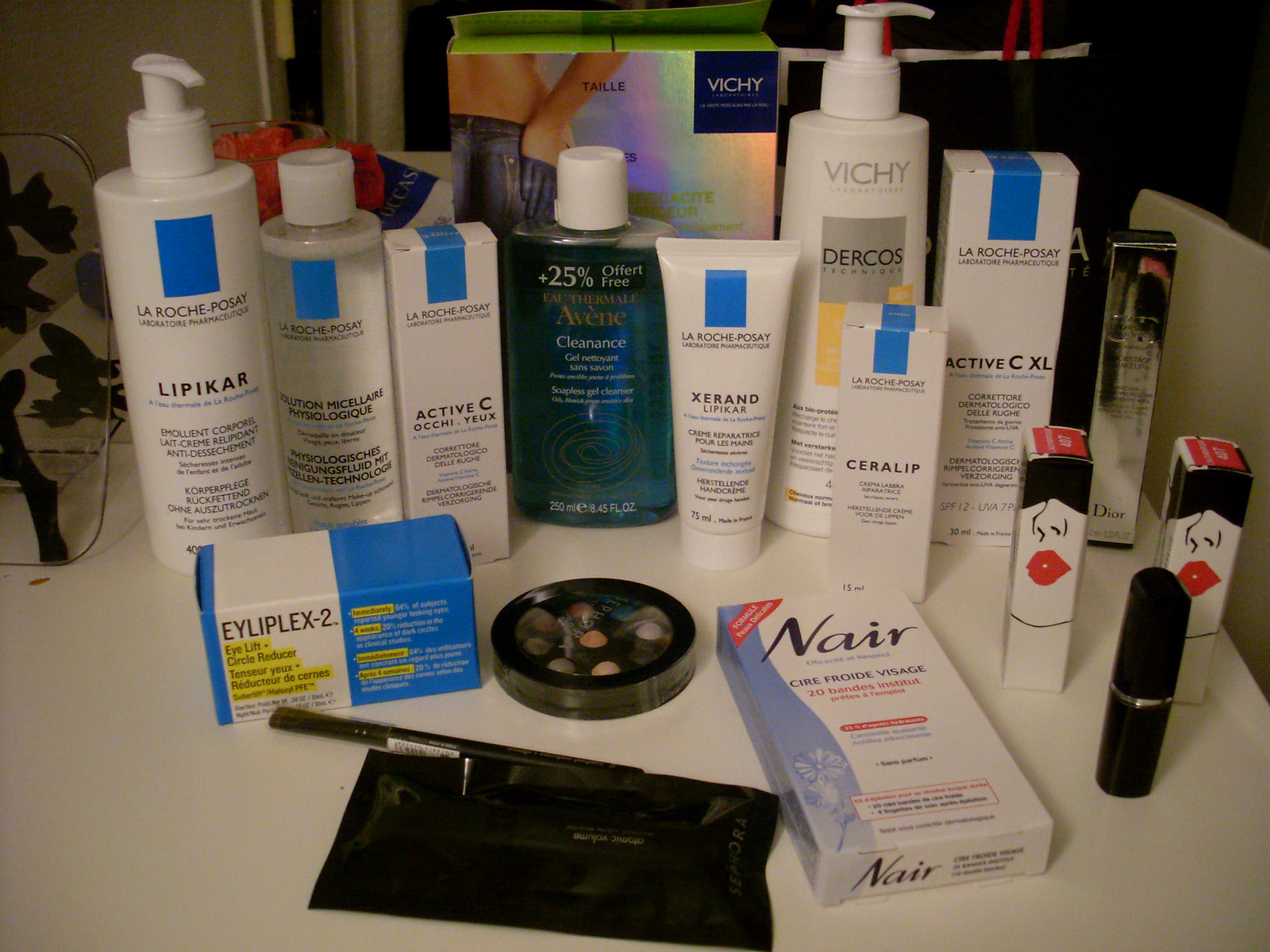The image showcases an assortment of skincare products neatly arranged on a white table, set against the backdrop of what appears to be a room. In the background, there is a box prominently featuring the brand "VICHY," with an image of a person showing their belly and wearing pants with a hand casually placed in the pocket. The arrangement begins on the left with a white bottle featuring a white pump, marked by a blue rectangle at the top, labeled "La Roche-Posay Lipikar." Next to it stands a clear bottle with a white cap, also bearing the blue square of La Roche-Posay, likely containing micellar water. 

This is followed by a white box with a blue rectangle, also from La Roche-Posay, labeled "Active C." Moving right, there is a blue bottle with a white cap, appearing to be some form of cleanser. Adjacent to it is another bottle from La Roche-Posay, similarly a cleanser, and next to it is another "Active C XL" product. To the bottom right, the scene includes two boxes of lipstick featuring black and white designs with pink lips, along with a black lipstick bottle. In the foreground, a box of Nair is visible. Additionally, there is a circular object with colored dots, possibly a lipstick palette, and a blue and white box labeled "Olaplex 2."